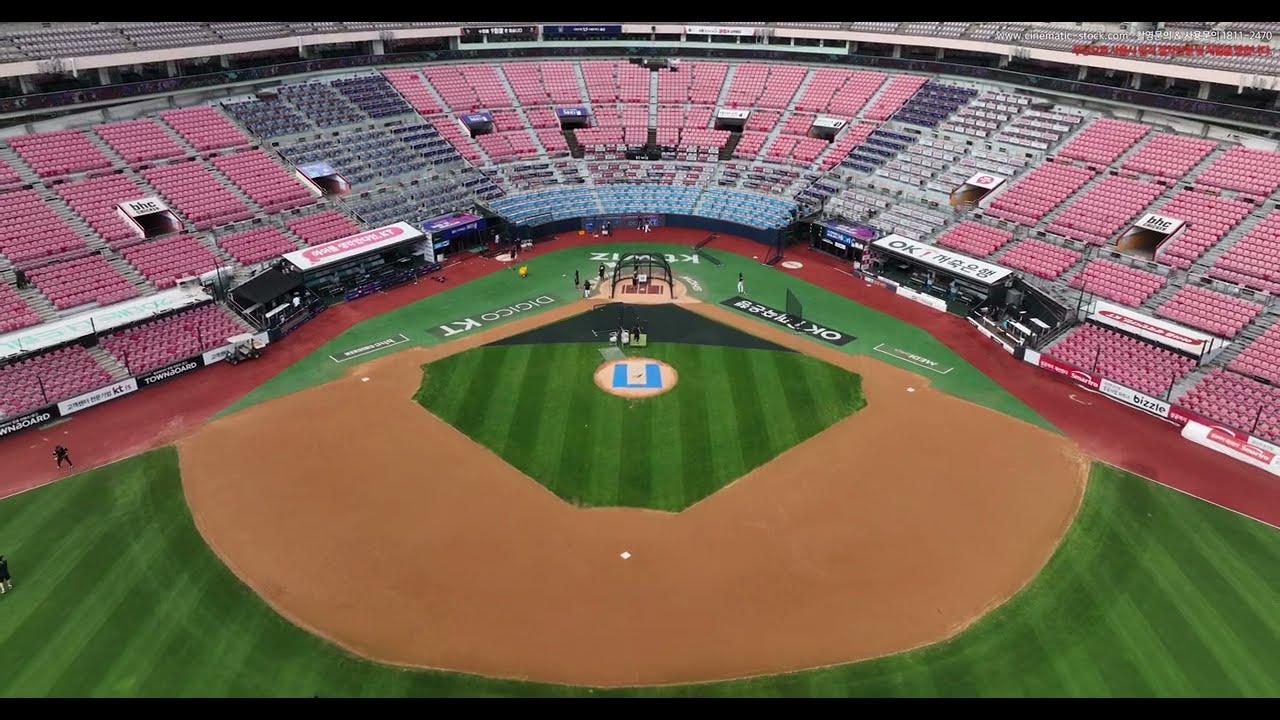The image is an aerial shot of a baseball stadium, framed by narrow black bands at the top and bottom. The central focus is the baseball diamond, with its infield dirt a distinctive brownish-red color. The grass is striped with alternating patches of lighter and darker green, presenting a striking contrast. The seating surrounding the field features predominantly red seats, with a notable blue section directly behind the catcher's area. 

Above the infield's sandy beige half-circle, a black batting cage and various ground markings for pitcher and batter position are visible. The field's perimeter is accented by a reddish-brown track, with light and dark green stripes extending across the grass in a visually pleasing pattern. Painted on the pitcher's mound is a prominent blue letter "U," and additional text, including "Digico KT," is visible along the baselines and various other parts of the field. The stadium's higher seating has black and light gray seats in addition to the red ones, and text such as "www.cinematic-stock.com" and Korean characters adorn the advertisement boards. The overall scene captures a vibrantly detailed and organized baseball field with noteworthy color contrasts and textual elements.